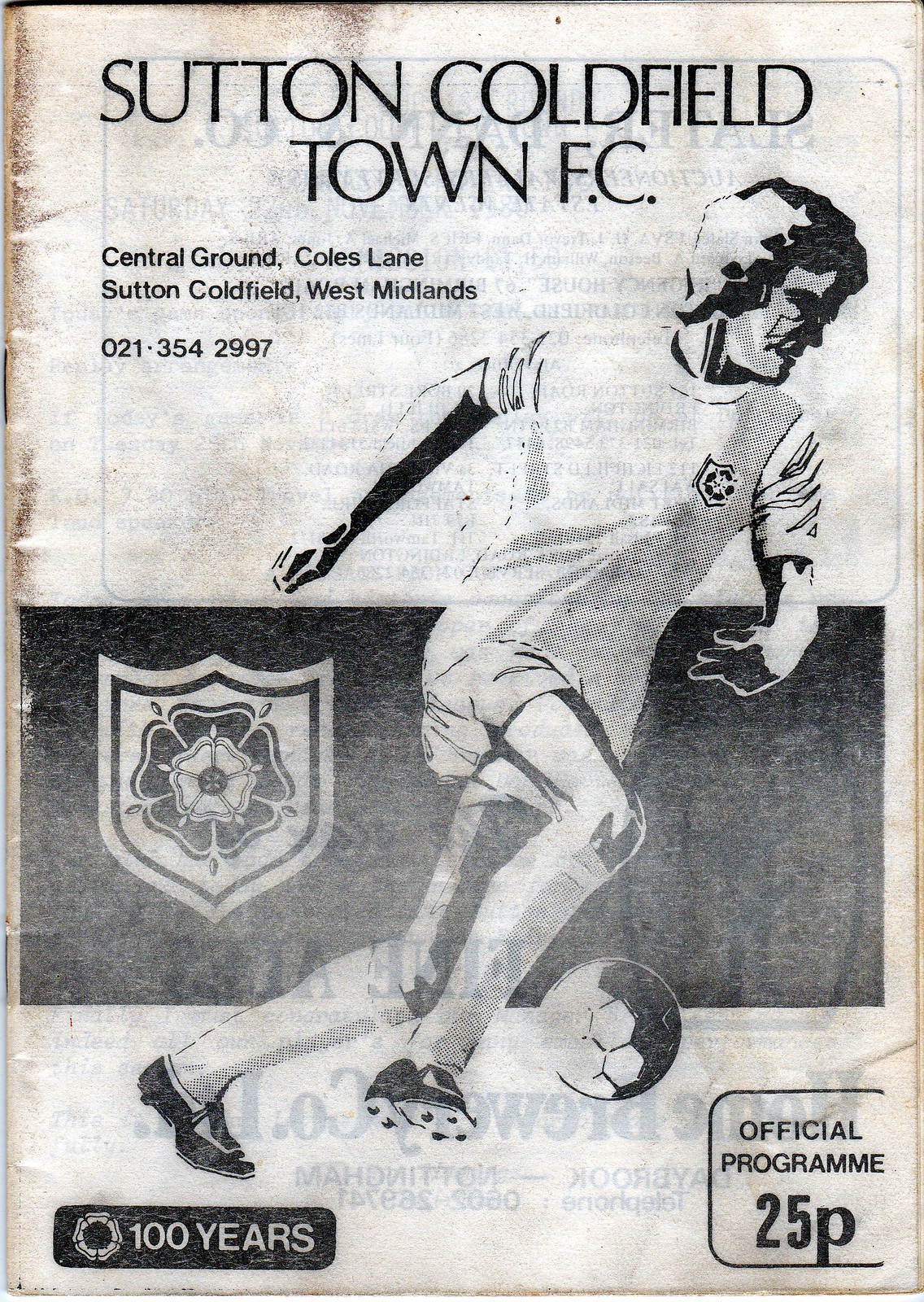Caption:

This vintage program showcases a black and white image of a soccer player in action, representing Sutton-Coldfield Town F.C. The top of the program provides essential details: "Sutton-Coldfield Town F.C., Central Ground, Coles Lane, Sutton Coldfield, West Midlands, 021-354-2997." A prominent black box at the bottom displays a shield with a floral design, commemorating the club's centennial celebration with the inscription "100 Years" on the left. On the right side of the box, it denotes "Official Program, 25P". The program’s age is evident from the bent, dirty, and browning paper, along with some fading ink, suggesting it as a cherished piece of history.